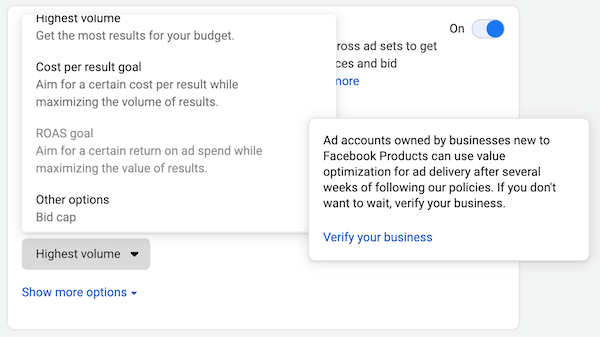This image is a screen capture of a website displaying multiple pop-up boxes. The background color is a very pale gray. The main interactive elements consist of three distinct pop-up boxes, each white with black text, alongside a gray button and a blue clickable link at the bottom.

In the background, in the top right corner, there is a small button toggled to the "on" position. This section includes partially visible text that appears to reference an advertisement setting, mentioning terms like "cross add sets," and "bid."

The largest pop-up box on the left side contains four main sections:
1. **Highest Volume**: "Get the most results for your budget."
2. **Cost per Result Goal**: "Aim for a certain cost per result while maximizing the volume of results."
3. **ROAS Goal**: This is grayed out, indicating it isn't selectable. The text reads, "Aim for a certain return on ad spend while maximizing the value of results."
4. **Other Options**: "Bid cap."

To the right of this primary pop-up is a smaller pop-up box. The text inside it reads:
"Ad accounts owned by businesses new to Facebook products can use value optimization for ad delivery after several weeks of following our policies. If you don't want to wait, verify your business." Below this text is a clickable link labeled "verify your business."

At the bottom of all these pop-ups, remnants of the original webpage are visible. There is a gray button labeled "Highest Volume" with a drop-down menu and a blue link labeled "Show more options" also with a drop-down menu.

Overall, the image captures a user interface focused on advertising options with descriptions and actions potentially related to setting up or optimizing ad campaigns.